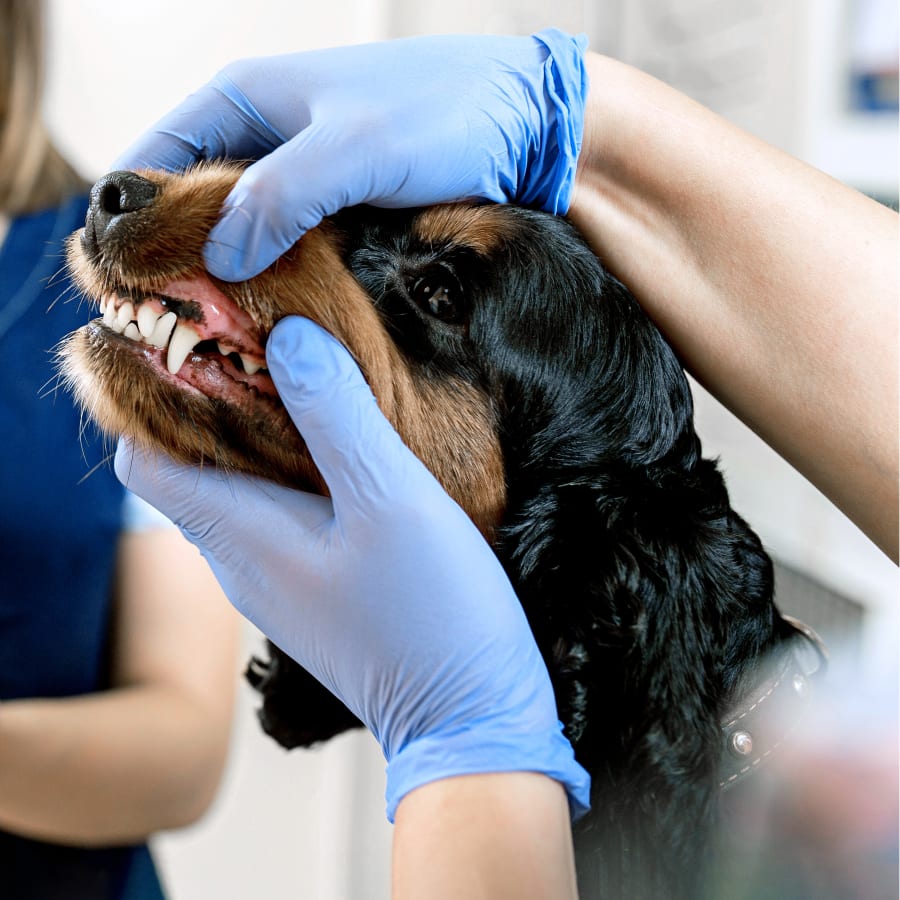In the picture, a small to medium-sized dog, primarily black with a light brown snout and brown eyebrows, is at a veterinarian's office. The focused image captures the dog's face, highlighting its brown eyes and healthy teeth with no visible plaque. A veterinarian, whose complete identity isn't visible, is seen wearing blue latex gloves, using one hand to lift the dog's upper lip and the other to support its chin, exposing the dog's teeth and gums for examination. In the blurred background, either an assistant or the dog's owner, dressed in blue scrubs and with blonde hair, stands by, likely ready to assist if needed. The dog's expression appears cooperative, if slightly uncertain, as it undergoes this check-up.